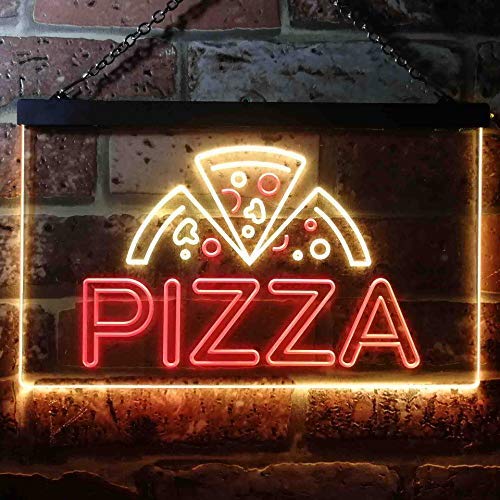This detailed square photograph captures a neon sign mounted on a richly textured brick wall. The wall itself is an intricate mosaic of deep red, gray, and orange bricks interspersed with light gray grout. At the center of the image, the neon sign hangs from a black chain beneath a black rectangular bar, likely made of metal. The sign's distinct feature is its vibrant lighting: "PIZZA" is prominently displayed in large, bright red neon letters at the bottom. Above the word "PIZZA," the sign showcases three outlined pizza slices in crisp white neon, accentuated with vivid red circles representing pepperoni, and additional white details hinting at mushrooms and cheese. The white neon piping gracefully outlines the slices, creating an appetizing and inviting glow. This hanging sign, potentially located inside or outside a pizza restaurant, emanates a classic, enticing feel against the backdrop of the richly colored brick wall.